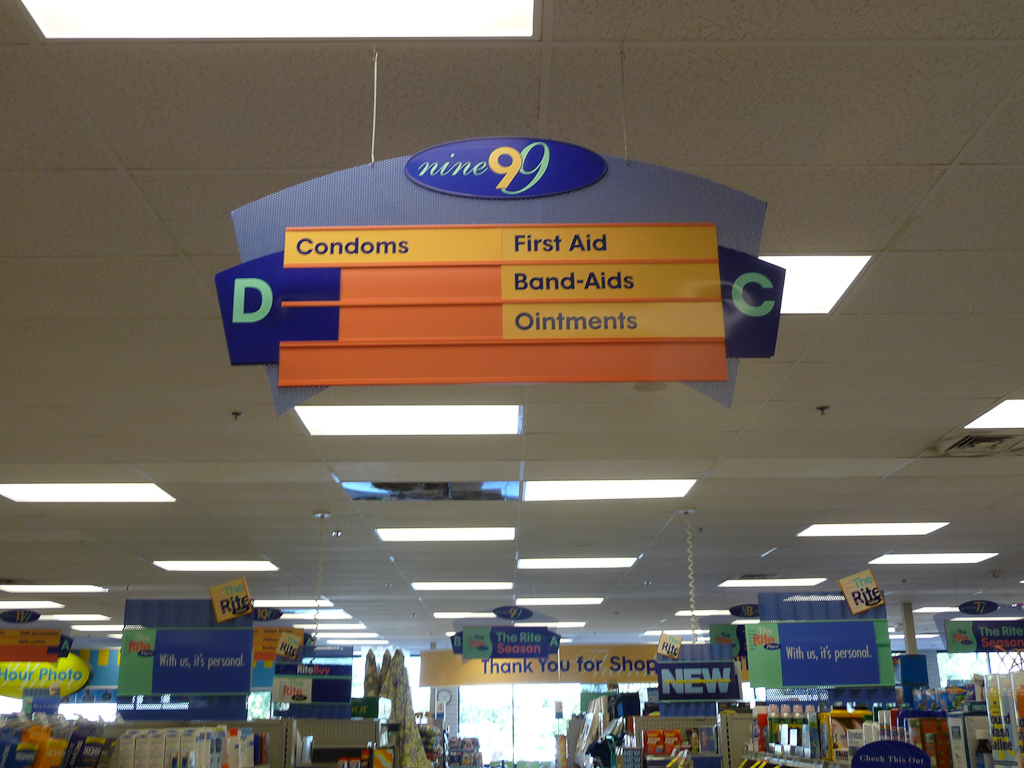This photograph captures an intricate sign hanging from the ceiling of a store, surrounded by various ceiling tiles and fluorescent light fixtures. The primary sign features a curved top and rectangular sides, adorned with an oval element. The oval showcases the word "nine" in cursive, accompanied by a yellow number nine and a larger, elegant blue number nine layered behind it. Below this prominent sign is an orange aisle indicator with blue extending tabs on either side, labeled "D" and "C," respectively. The "D" section highlights 'condoms' on a yellow background with blue text, while the "C" section lists 'first aid, band-aids, and ointments.' At the bottom corners of the image, additional signs emphasize customer care messages, reading "With us, it's personal" and "Thank you for shopping" further in the background. The ceiling is detailed with neatly arranged tiles and integrated fluorescent lights, contributing to the well-lit ambiance of the store.